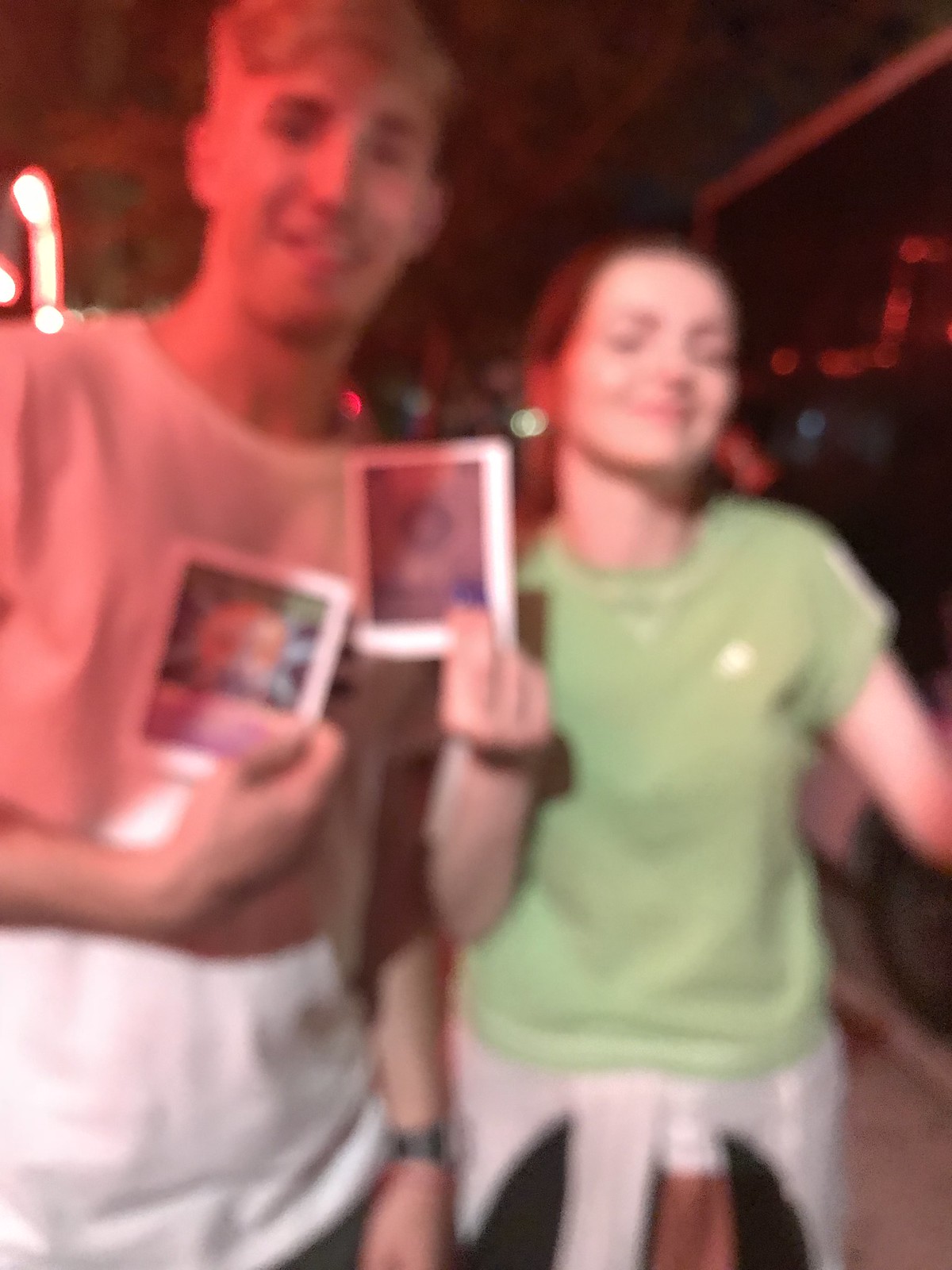In this vertically oriented, rectangular image, two young individuals pose facing the camera amidst a blurry and grainy atmosphere that evokes a sense of nostalgia or candidness. We see them from the thighs up against a backdrop punctuated by soft, ambient lighting, hinting at an indoor setting bathed in faint fluorescence from the upper left corner.

On the right side of the frame stands a young woman with strikingly fair skin and red hair pulled back from her face. She is clad in a pale green crewneck t-shirt, its gentle hue contrasting with the cream-colored sweatshirt or jacket tied around her waist. Below, she wears dark pants or shorts. In her right hand, she holds a photograph or card, though the details are indistinct due to the image’s graininess.

To her left, a noticeably taller young man stands confidently in a white crewneck t-shirt. His left arm hangs down naturally, adorned with a dark wristwatch, while his right hand is raised, displaying another card or piece of paper similar to the one the young woman holds. The image is vibrant despite its blurred lines, capturing a moment suspended in time against the enveloping shadows in the background.